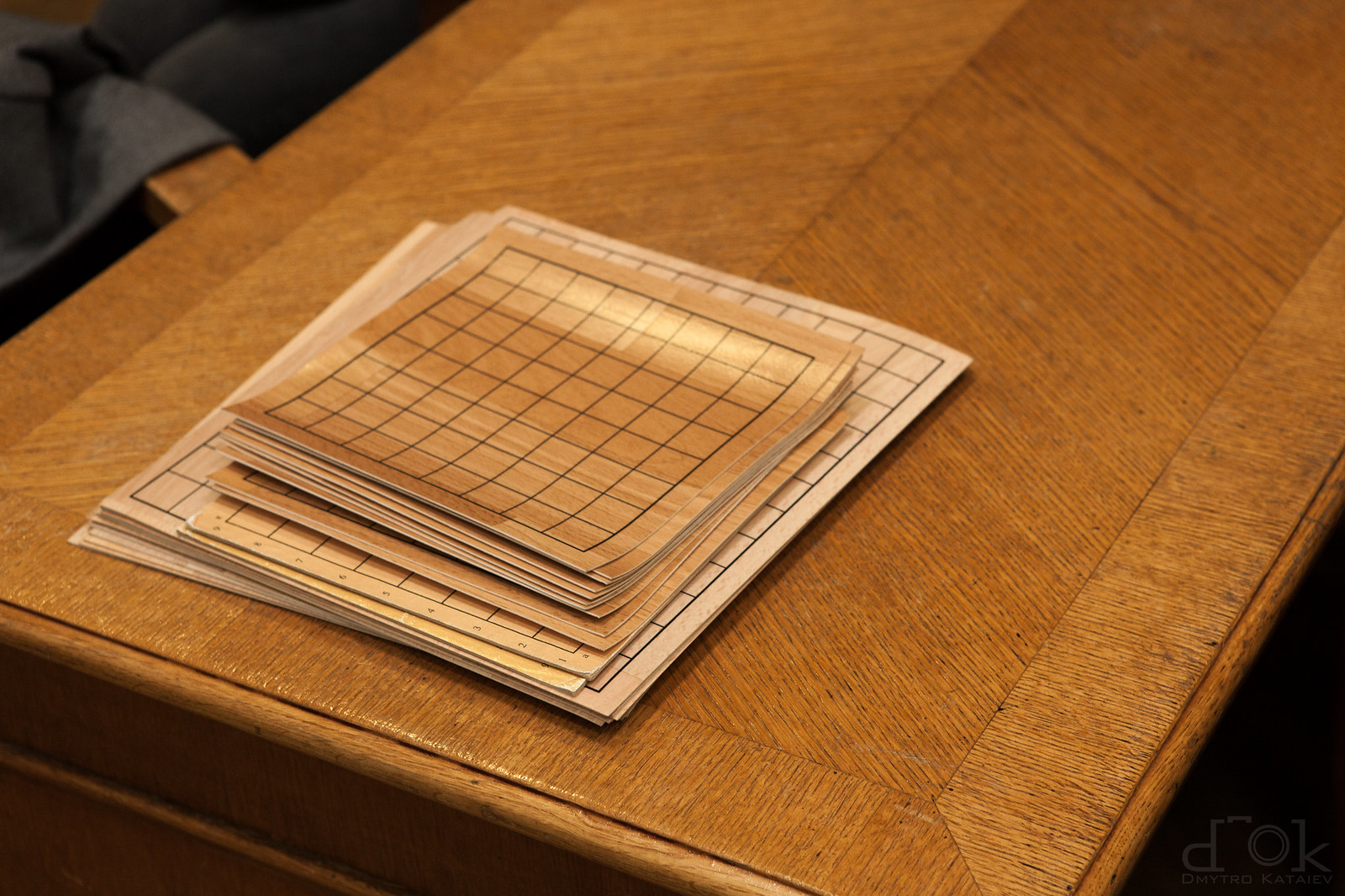This indoor color photograph focuses on a rectangular coffee table with a natural wood finish, extending from the lower left to the upper right corner out of the frame. Situated at the end of the table, towards the very edge of one of the short sides, is a stack of thin laminate sheets. These sheets, resembling either paper or fabric, feature a crisscross grid pattern on one side. They appear to be dark brown with black grids and range in color from medium brown to blonde, matching the wood grain of the table beneath them. The underlying table, possibly a cupboard or chest, also has pieces angled at various corners, adding to its textured appearance. In the upper left corner, a wooden chair with a black or blue cloth draped over it is partially visible. The remaining corners of the image are dark and there is no text present, maintaining a clean and sharp focus on the arrangement.